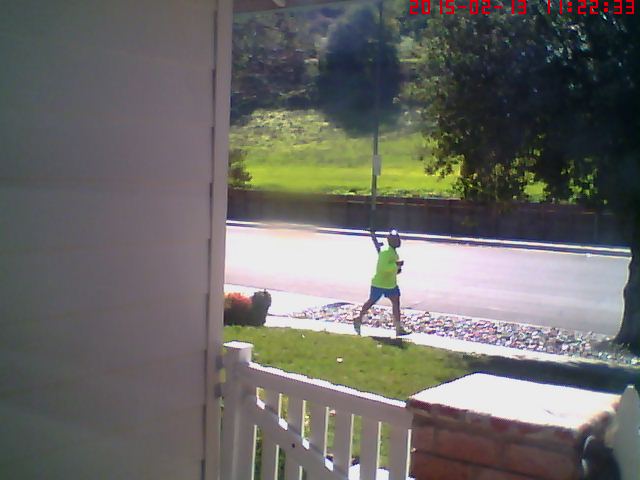A photograph taken from the front porch of a charming white-painted home with shingled siding captures a serene suburban scene. The porch features a distinctive red brick pillar in the center, flanked by two pristine white-painted wooden gates. Stepping down from the porch, a neatly maintained green front lawn leads to a sidewalk. On the sidewalk, a person in motion catches the eye—dressed in blue shorts and a long-sleeved neon yellow sports shirt, their dark skin suggests they are African American, and their bald head and white tennis shoes with socks further detail their appearance.

As the person jogs past, they are poised to run beneath a large, leafy tree that stands beyond the sidewalk within an area landscaped with rocks and pebbles. The scene extends across a quiet road void of traffic, leading to a brown fence that borders a grassy incline adorned with more trees. The photograph captures a moment of daily life in a peaceful neighborhood, emphasizing the blend of natural beauty and human activity.